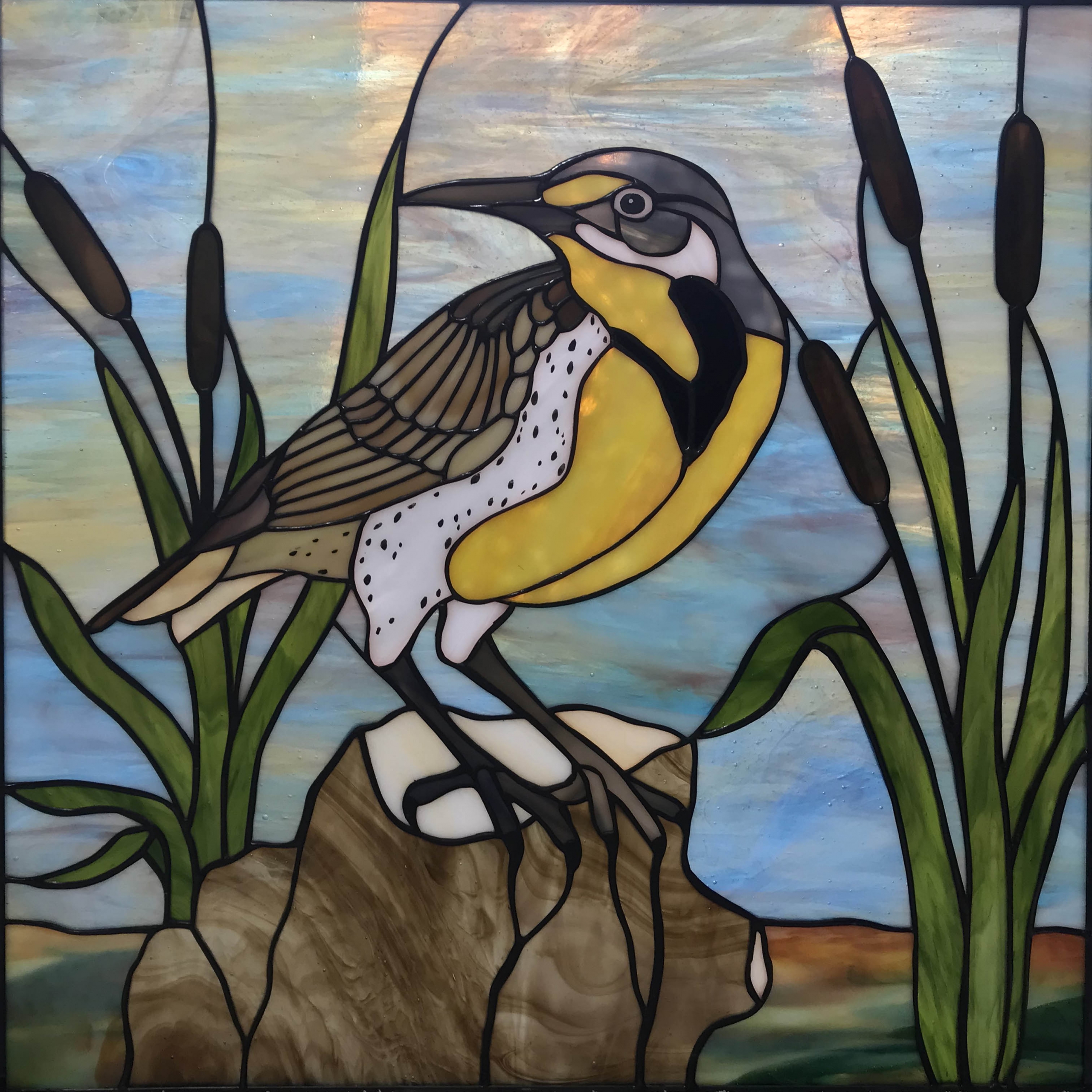This detailed stained glass art piece depicts a vibrant bird standing on a tree stump. The bird's intricate design features a primarily yellow breast accented by a black section, a gray head with a yellow patch, and a white beak tinged with brown. Its body also showcases a white area adorned with dark speckles and brown feathers extending down its back. The bird's legs and talons are dark brown, gripping the tree stump beneath it. Surrounding the bird are green willow leaves and brown-tipped pods, adding a naturalistic touch to the scene. The background is a beautiful blend of blue hues, infused with streaks of brown, yellow, and white, creating a picturesque sky that enhances the stained glass effect. The tree stump, with its brown and white tones, and the gray and brown ground, complete this stunning and detailed piece.